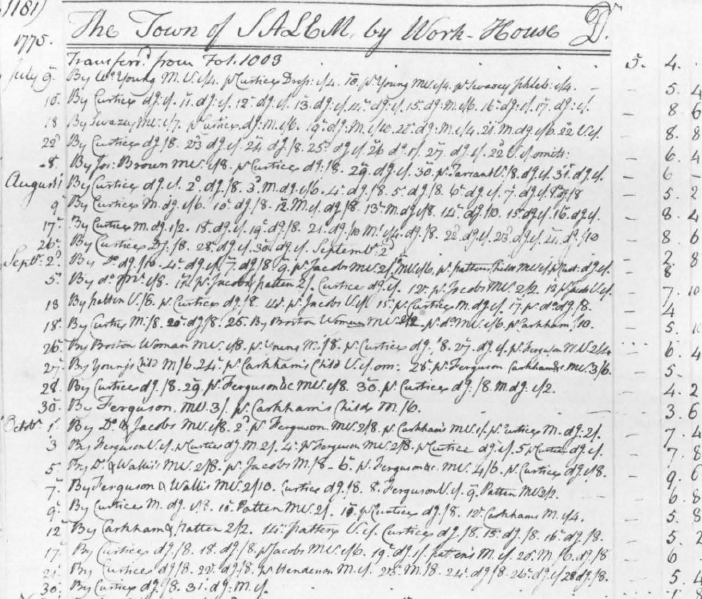The image showcases a historical record dating back to 1775, appearing to be a handwritten manifest. The document features a neatly cursive title that seemingly reads, "The Town of Sallby Work-House," though parts of the title and some handwriting are difficult to decipher due to the ornate cursive script. The left-hand column lists dates starting from July 9th, progressing through various entries on July 10th, 18th, 22nd, 28th, and then moving through August, September, and finally October 30th. Each date is accompanied by handwritten notations that span across multiple columns, some of which appear to be cut off. Additionally, there's an inscription at the top of the main text stating, "Transfer from FOL103 by," followed by an unreadable name. The paper appears to be an official document from the 1700s, potentially a manifest or a municipal record, meticulously recorded in cursive.